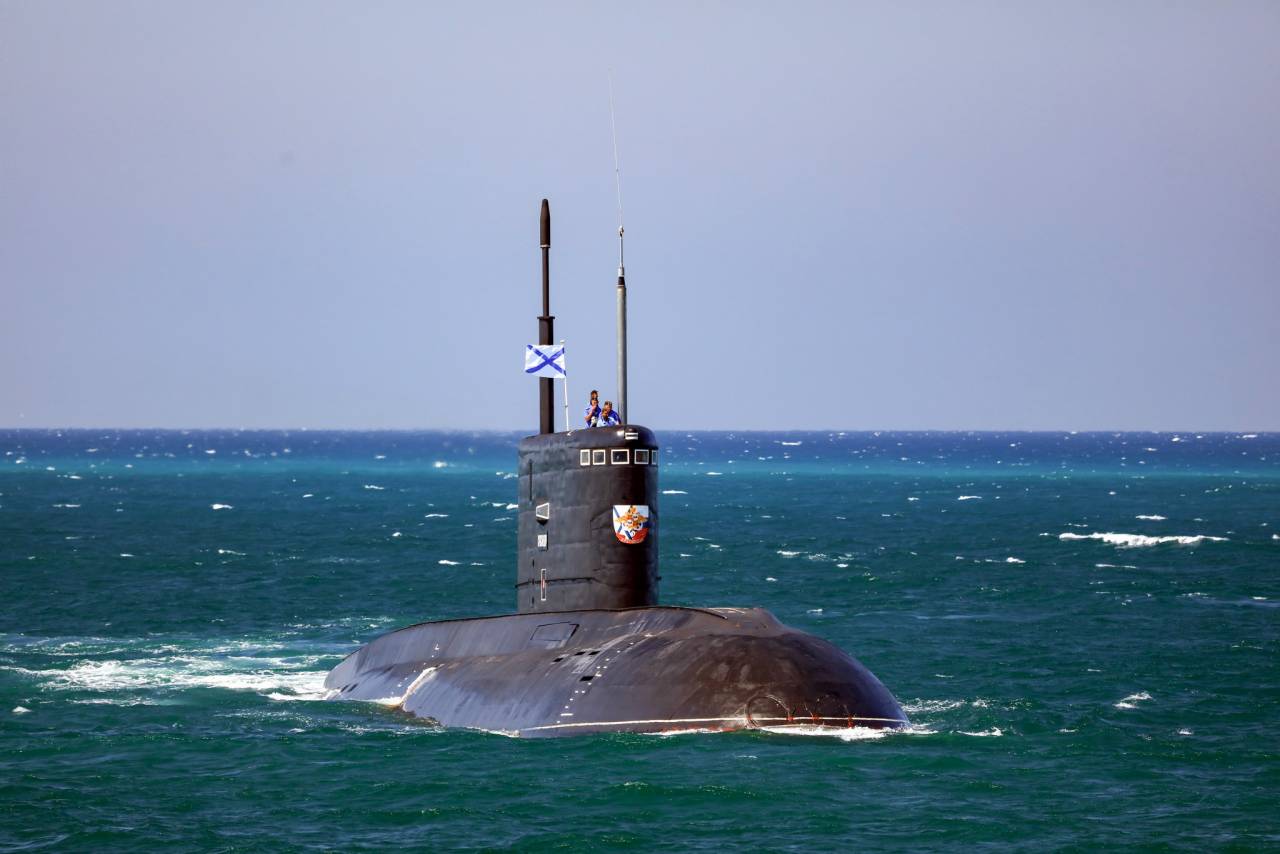In this daytime photograph, a grey-black submarine partially surfaces on greenish water, revealing its top structure with two distinct towers, one black and the other greyish-white. At the forefront of the submarine’s conning tower, a shield with a red, blue, and yellow design is visible. A flag with a blue X on a white field flutters above, and another smaller flag with a blend of white, yellow, and a bit of red can be seen below the windows, which resemble white squares. Two individuals, possibly wearing blue shirts, are seen waving from the hatch area, surrounded by several windows and footholds on the submarine’s exterior. The scene is serene with water ripples visible on the horizon, enhancing the image's tranquil maritime setting.